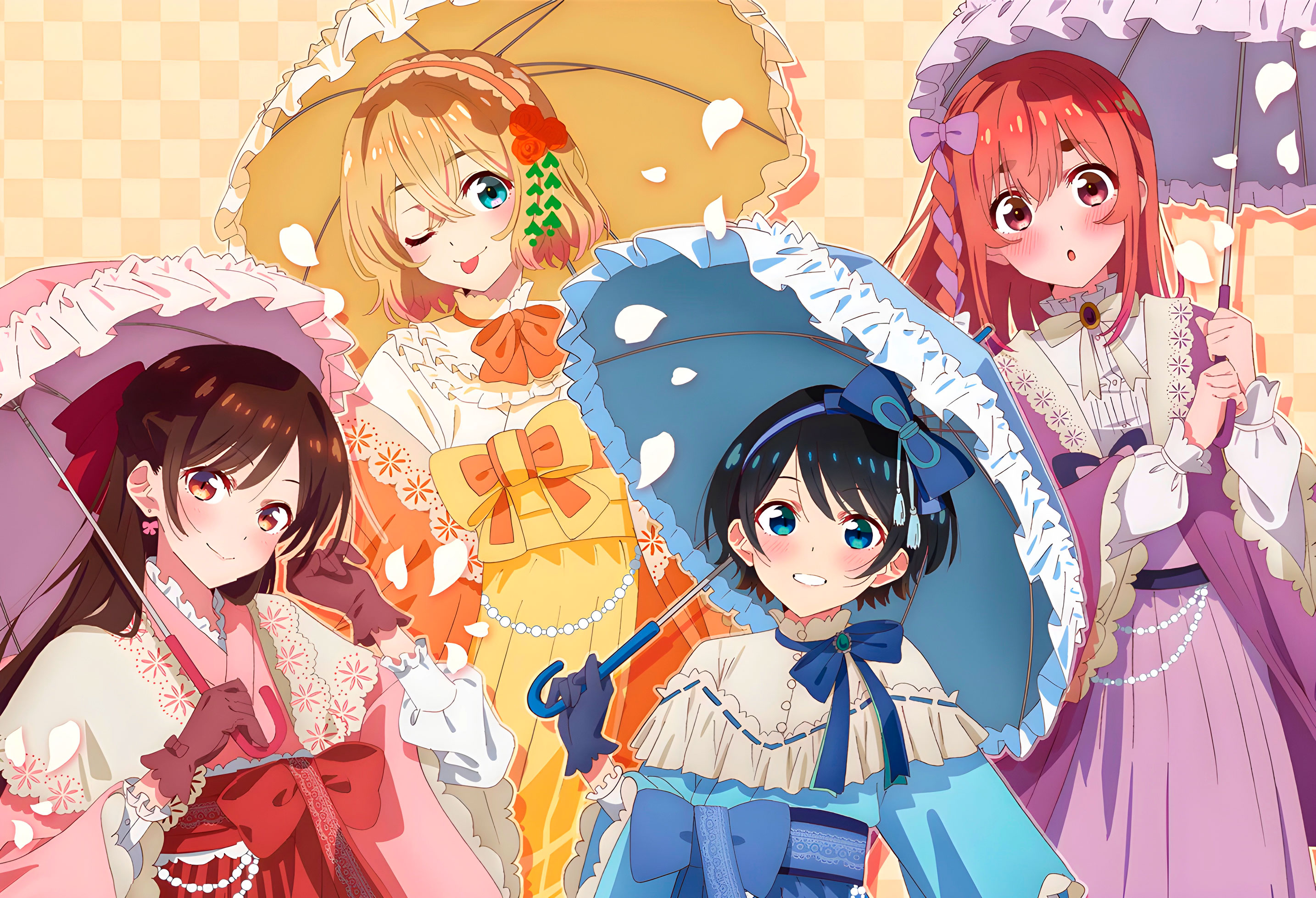This is a highly detailed, full-color drawing of four anime or manga-style women set against a yellow and white checkerboard background. Each woman wields a distinctively colored umbrella that complements her formal, possibly 18th-century-inspired attire, each adorned with intricate bows and embellishments.

Starting from the left, the first woman has striking red hair and is dressed in a red dress accented with a bow and pearls at the waist. She holds a pink umbrella with a lacy lighter pink center and wears matching pink gloves. She has a surprised expression on her face.

Next to her is a woman in various shades of blue. She has short black hair and wears a dress featuring a blue and white combination, accentuated by blue bows at the neck, waist, and in her hair, with tassels hanging from the bow. She carries a blue and white lace parasol with a blue handle and has a neutral, everyday expression.

Behind them is a woman dressed in a mix of darker and lighter purples with white accents. She holds a purple umbrella and has reddish hair. She appears composed and content.

Furthest to the right stands a blonde woman in an orange dress with a prominently large orange and yellow bow. She wields an orange umbrella and has a playful expression, winking and sticking her tongue out.

Each character's distinctive look, attire, and expression contribute to a vibrant and engaging image.